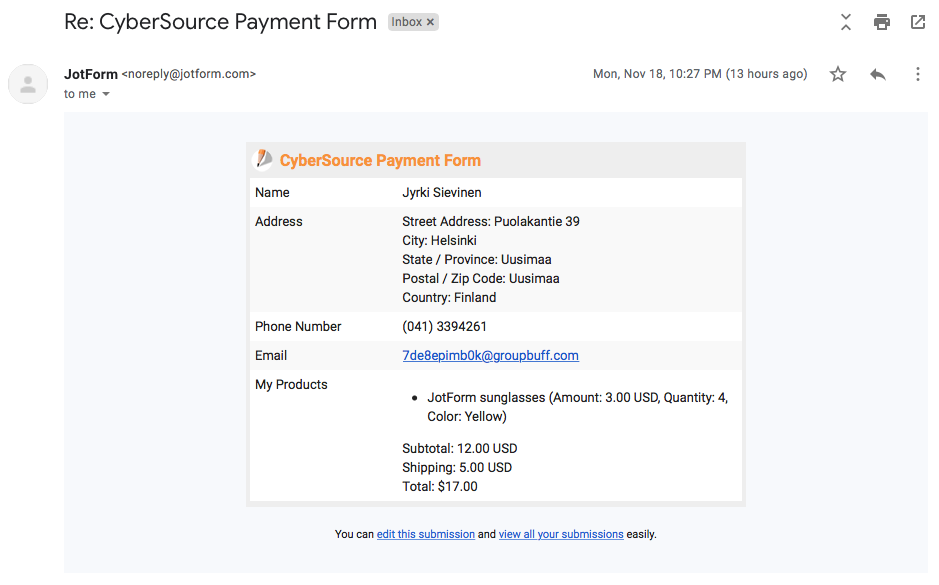Here is a cleaned-up and detailed caption for the image:

The image is a screenshot of a web page titled "RE: Cyber Source Payment Form." In the top left corner, the title is clearly stated, while to its right, a gray box labeled "Inbox" is visible. In the top right corner, there are two icons—one resembling a printer and another depicting a box with an upward-pointing arrow. Just below, there's a circular icon with a generic profile picture, followed by the text "JotForm," and the email address "NoReply@JotForm.com." To the right of this, a dropdown menu shows the recipient as "To Me." Further to the right, the date and time are displayed: "Monday, November 18th, 10:27 PM, 18 hours ago." Adjacent to these details are a star icon and a left-pointing arrow.

Beneath the header section, the main content sits against a gray background. At the top, an orange square prominently displays the title "Cyber Source Payment Form." The form contains personal information for an individual named Jyrki Sluvin, including the address "Polanki 39, Helsinki, Jysmäe, Jysmäe, Finland," along with a phone number "041-339-4261" and email "7D8EPIMBOK@groupbluff.com." The form also lists purchased products: "JotForm Sunglasses" with details—amount: $3, quantity: 4, color: yellow. The cost breakdown shows a subtotal of $12 USD, shipping at $5 USD, for a total of $17 USD.